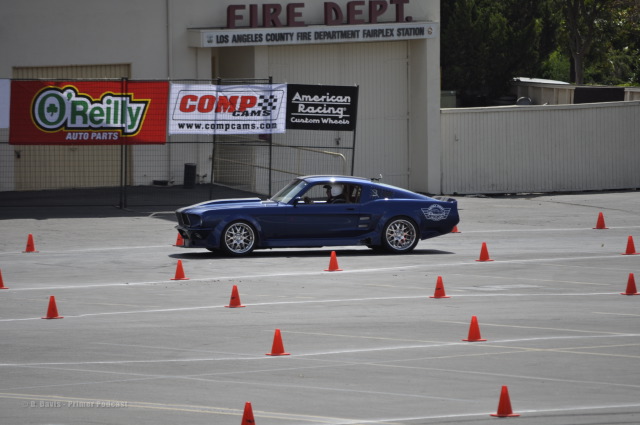The image depicts a driving obstacle course featuring a sleek blue sports car, likely a Mustang model, designed with vintage elements reminiscent of 70s or 80s Mustangs. The setting appears to be a concrete platform or a parking lot, lined parallel with multiple orange cones creating a detailed and structured course. In the driver's seat, there is an individual wearing a white helmet, suggesting that this may be a training session for racing. Positioned in front of the Los Angeles County Fire Department Fairplex Station, the background includes a large white warehouse and a chain-link fence adorned with banners from sponsors such as O'Reilly Auto Parts, COMP Cams, www.compcams.com, and American Racing Custom Wheels. The well-organized layout of cones and prominent branding hints at a professional training environment possibly associated with competitive racing or advanced driving instruction.